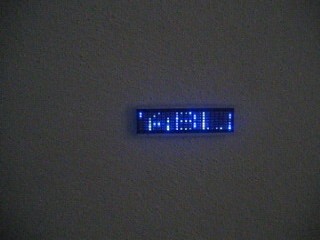The image features a small, rectangular sign affixed to a white wall. The sign is black with a pixelated, white text that has a faint bluish hue. The visible portion of the text includes the letters "A", "B", "L", and partial letters that suggest the word "table." The photograph is taken in a low-light setting, accentuating the contrast between the sign and its background. The surrounding darkness adds a dramatic effect to the scene, highlighting the sign's distinct features against the white wall.